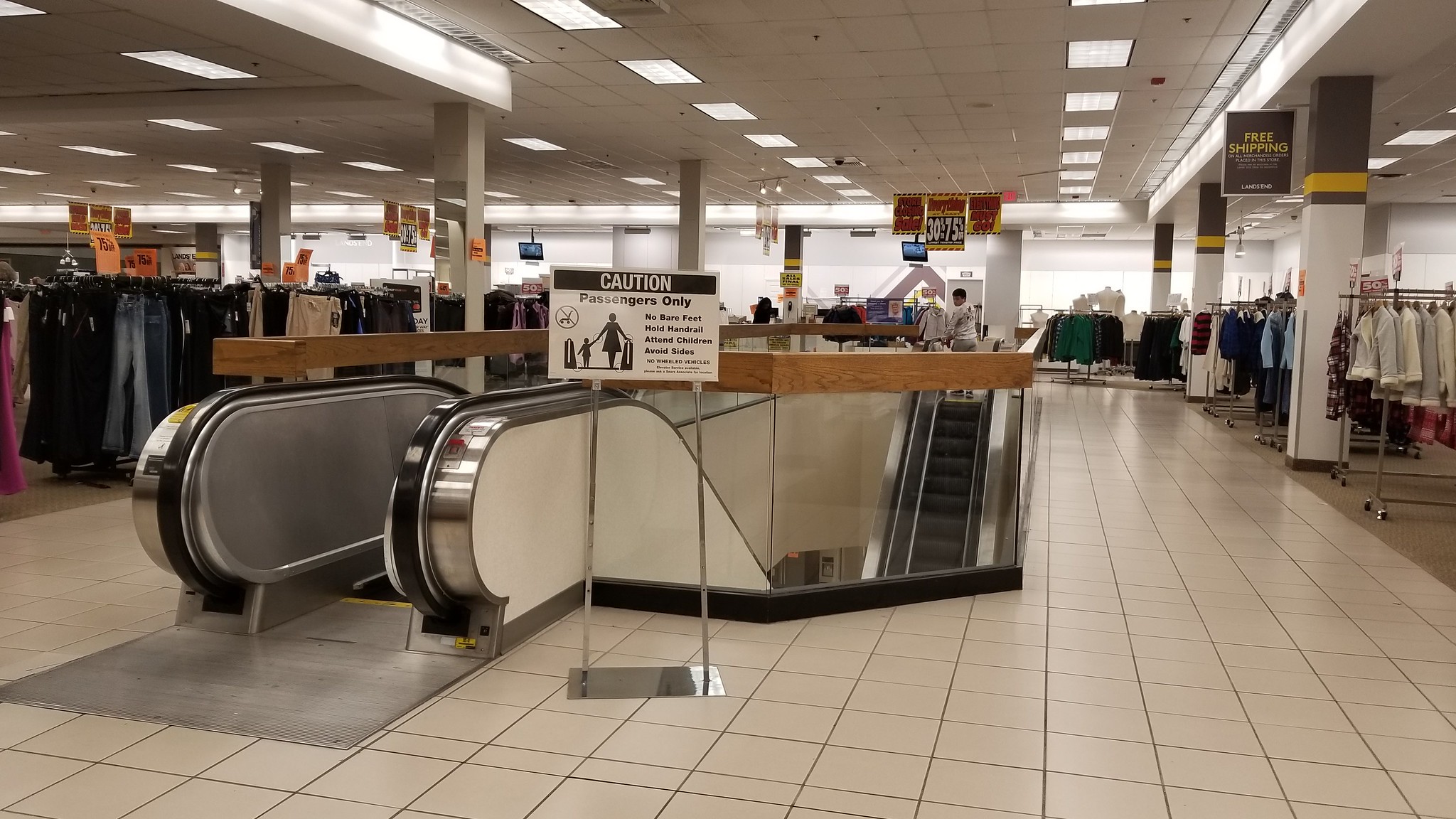The color photograph, taken in a wide landscape orientation, captures the interior of an upper-level floor within what appears to be a department store, specifically showcasing a clothing section. Dominating the center of the image are two escalators—one going up and one going down—emphasizing that this is indeed at least one level above the ground floor. In front of the escalators stands a metal sign with two vertical poles, stating "Passengers Only" in black text, accompanied by an illustration depicting a mother and child using the escalator safely by holding the handrail.

Surrounding the escalators is a mix of flooring materials: tan-colored carpet covering the clothing areas and off-white ceramic tiles where the escalators are situated. The well-lit environment features basic fluorescent lighting and a drop-style tiled ceiling with various hanging signs, including one on the right side with a black background and yellow text that reads "Free Shipping." The clothing section around the escalators is filled with garments on hangers, with trousers visible on the left and various shirts and jackets on the right. The overall scene provides a detailed glimpse into the everyday layout and signage of a modern department store.